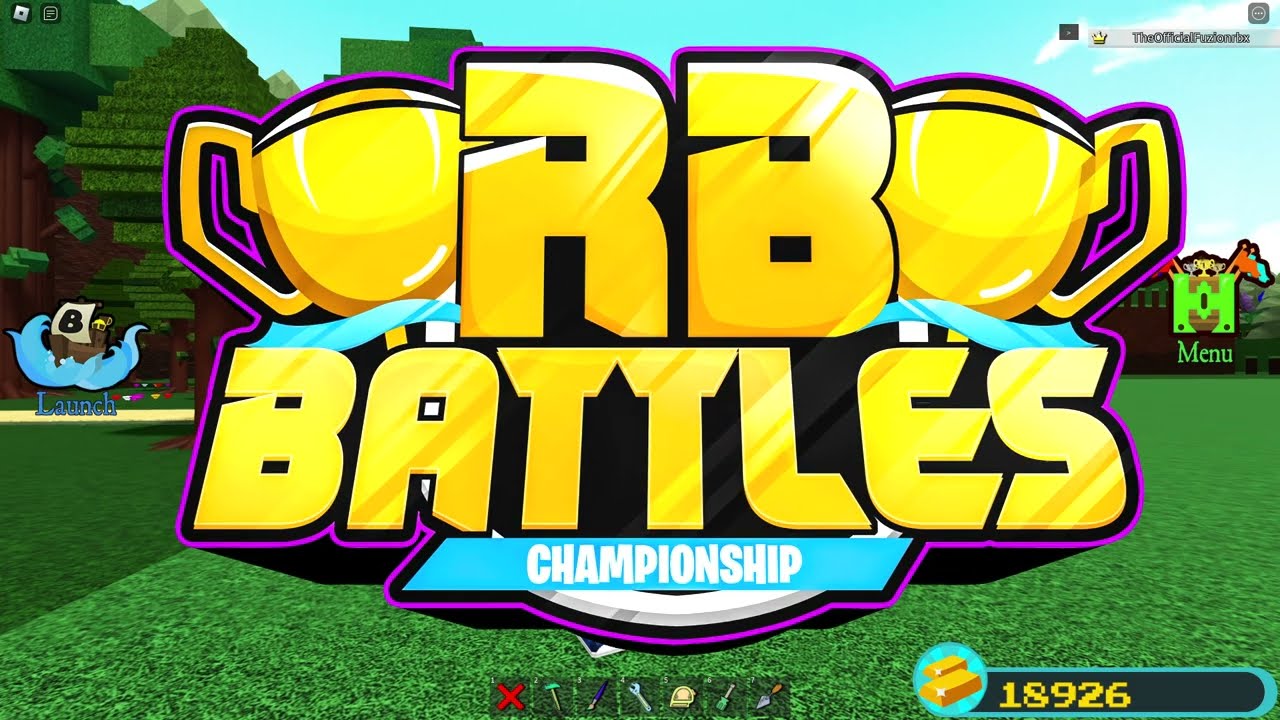The screenshot captures a vibrant moment from a video game, displaying the opening sequence of the RB Battles Championship. At the center of the image, large text is prominently featured with "RB" and "Battles" written in shiny gold, encased in black and purple outlines, and flanked by two large gold trophies. The word "Championship" is displayed on a blue banner in white text. These elements are set against a pixelated, Minecraft-style background featuring a field of lush green grass, block-shaped trees on the sides, and a strip of bright blue sky at the top. Additional game interface details are scattered throughout the image: an icon labeled "Launch" with a little boat bearing the letter 'B', and another icon labeled "Menu" with a green box and flags. At the bottom center, various game icons are visible, and in the bottom right corner, the score of 18,926 is displayed beside some gold bars. Meanwhile, in the top right corner, the text "official Fusion RBX" is clearly marked.